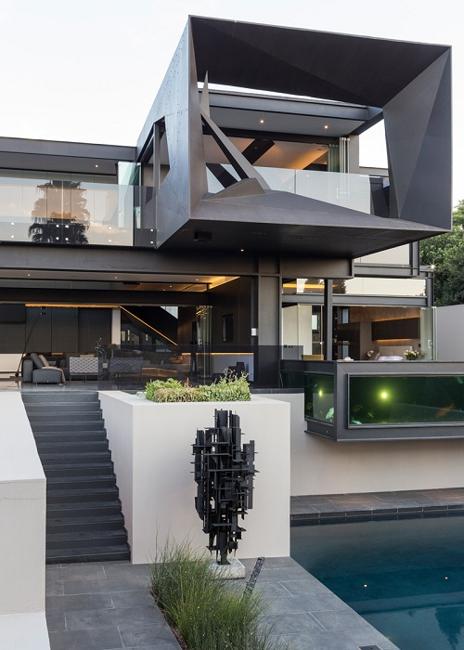The photo depicts an ultra-modern, minimalistic, and uniquely designed home with striking geometric architecture. The home features an abundance of linear elements and large, open windows, giving it a transparent appearance. The lower right side of the image showcases a pool or pond with a surrounding gray stone walking area and a modern sculpture composed of intersecting rectangles and squares. To the left, there are stairs leading up to an outdoor lounging area. A large metallic structure, resembling a balcony or overhang, extends around the white balcony, adding to the home's modernist aesthetic. The house itself has a prominent silver and white color scheme, with floor-to-ceiling windows reflecting a clear blue sky and nearby trees. Various green lights and artistic pieces are visible within and around the residence, emphasizing its unique and contemporary style. The setting likely suggests the home is situated in a picturesque location, possibly in America.